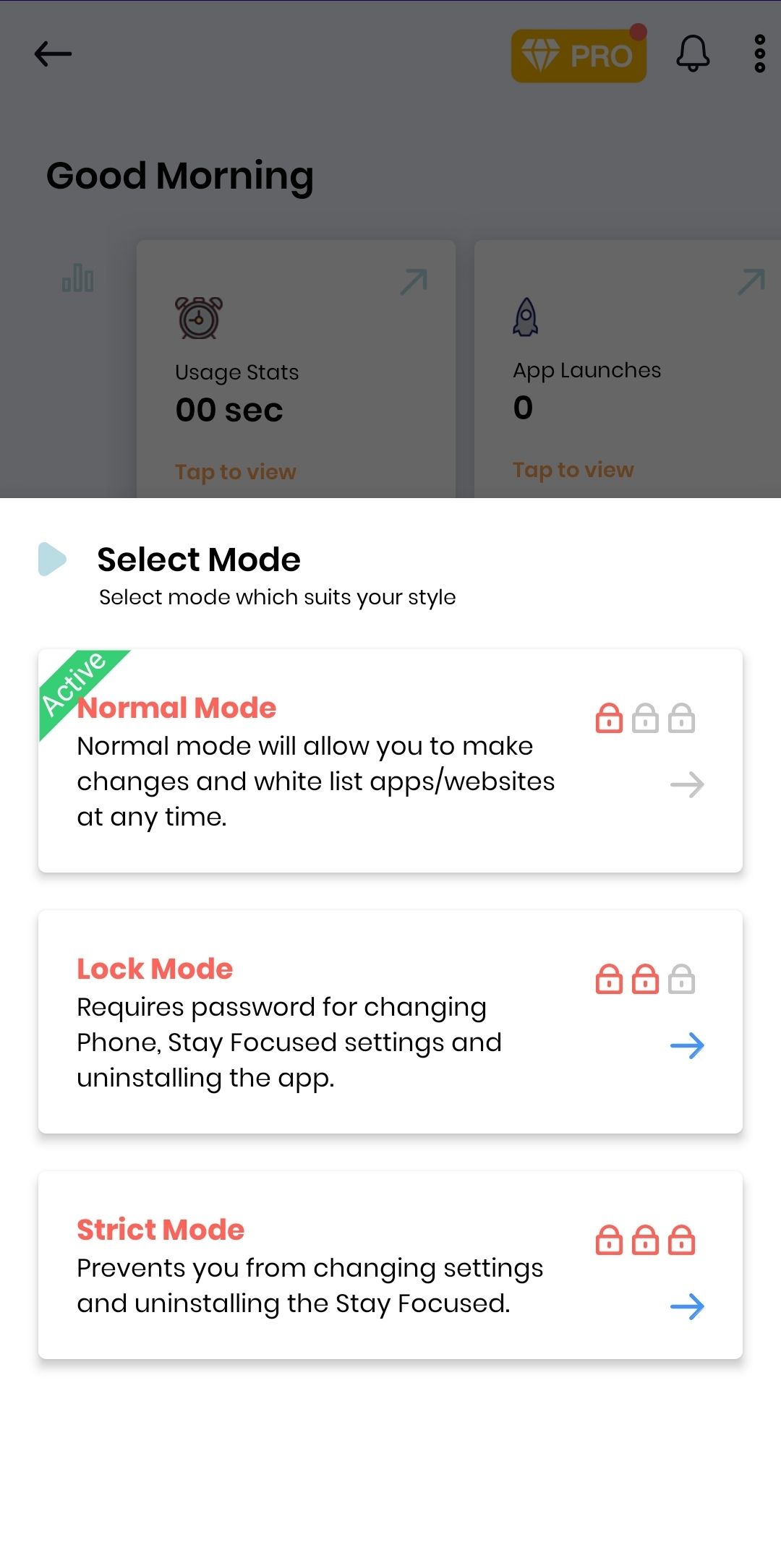This screenshot depicts a settings selection page from a mobile application. The photo itself has a portrait orientation and a seamless border, signifying it was likely captured on a smartphone. At the top of the interface, there's a long, rectangular gray box extending across the landscape orientation, suggesting it highlights key information.

Within this gray box, on the top left, there's a left-facing arrow for navigation, followed by a yellow box with a white diamond inside labeled "Pro". Adjacent to it, there's a red dot indicating a notification. Further to the right, you see a bell icon (likely for alerts) and a vertical ellipsis of three dots suggesting additional options.

Below this header, in bold black text, "Good Morning" is displayed, next to a graph or a graphic indicator. Just beneath, a white box labeled "Usage Stats" shows a clock icon and a text indicating "0 seconds", implying no recent activity. Another section below uses a rocket icon and states "App Launches: 0".

Following these statistics, there's another white section titled "Select Mode" in black font, with the instruction "Select the mode which suits your style". Below this, three white, long, rectangular boxes denote different modes:

1. **Normal Mode** - accompanied by a single lock icon.
2. **Lock Mode** - indicated by two lock icons.
3. **Strict Mode** - represented with three lock icons.

The current active mode, "Normal Mode," is highlighted with a green banner at the top left, featuring white font that reads "Active."